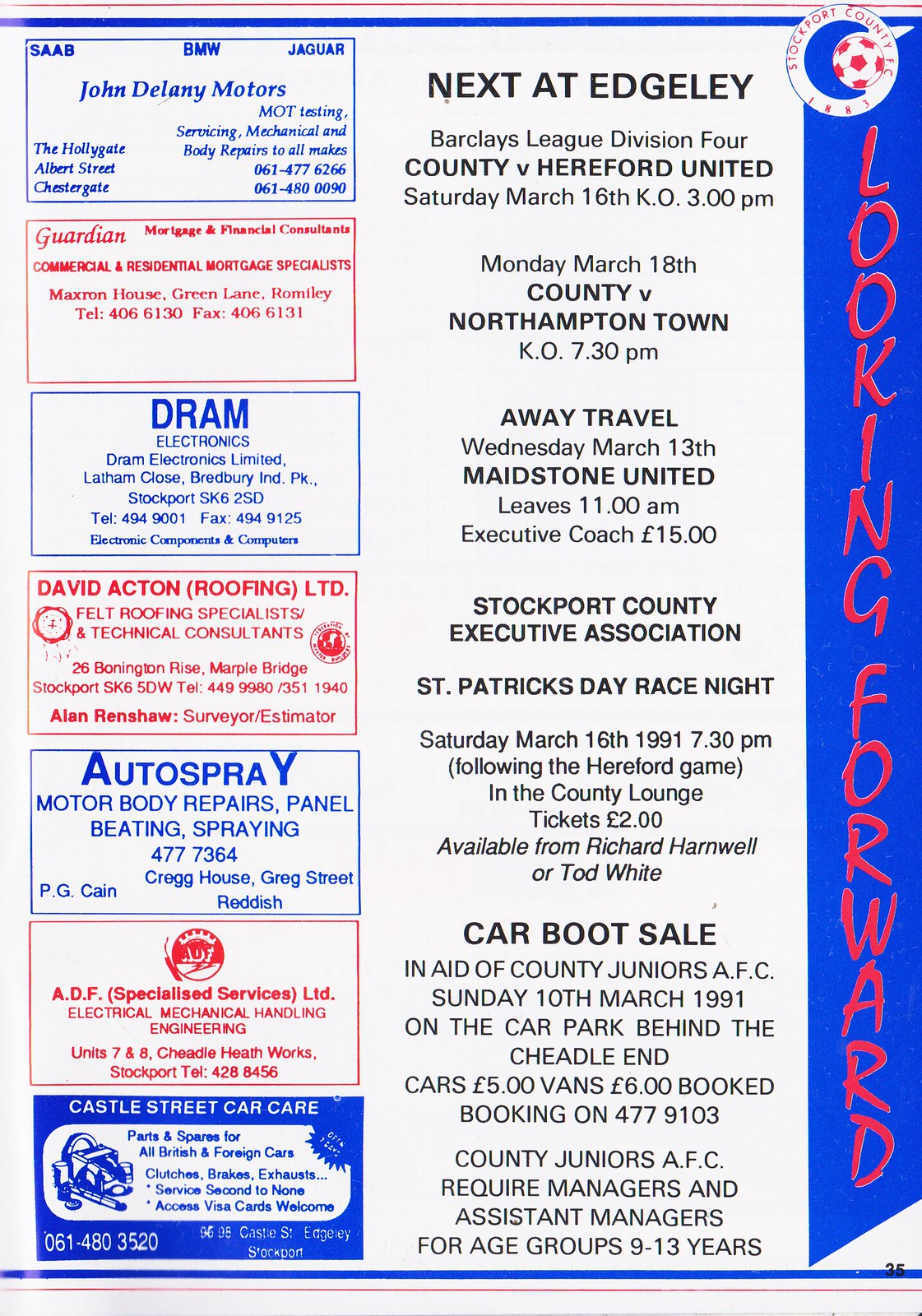The image is an advertisement poster with a white background and blue and red text. The left side of the image features seven business card-sized ads with alternating blue and red colors and fonts: John Delaney Motors, Guardian Mortgage and Financial Consultants, DRAM Electronics, David Action Roofing LTD, Auto Spray, ADF Specialized Services LTD, and Castle Street Car Care. Alongside these ads, it announces upcoming events at Edgley Park:

- Barclays League Division 4 match: County vs. Hereford United on Saturday, March 16th at 3 p.m.
- County vs. Northampton Town on Monday, March 18th at 7:30 p.m.
- Away travel to Maidstone United on Wednesday, March 13th, with the executive coach leaving at 11 a.m. for £15.

Additionally, there's a St. Patrick's Day Race Night on Saturday, March 16, 1991, at 7:30 p.m. following the Hereford game in the County Lounge, with tickets available for £2. There is also a car boot sale in aid of County Juniors AFC on Sunday, March 10, 1991, at the car park behind the Cheetah Land, with cars costing £5 and books £6. The County Juniors AFC is also recruiting managers and assistant managers for the 9 to 13 age groups.

On the right side of the image, in a vertical blue section with red font, it states, "Looking Forward," providing a comprehensive overview of the listed events.